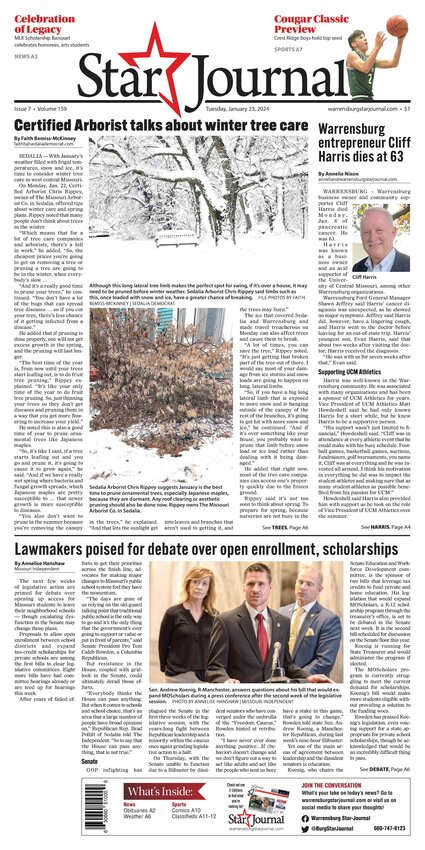The screenshot depicts a desktop capture of a newspaper page from the "Star Journal." The page features several articles and images. The primary headlines include:

1. "Celebration of Legacy: Cougar Classic Preview"
2. "Certified Arborist Talks About Winter Tree Care" accompanied by an image of a tree in winter.
3. "Warrensburg Entrepreneur Cliff Harris Dies at 63" with a photograph of Cliff Harris. The article provides a brief obituary mentioning that Cliff Harris passed away on a Monday in January, although the exact date is unclear.
4. "Lawmakers Poised for Debate Over Open Enrollment Scholarships," which includes a picture of several lawmakers, possibly high-ranking government officials.

Towards the bottom of the page, there are various advertisements, including a subscription barcode for the "Star Journal." The content is dense, with a significant amount of small text that is difficult to read in detail.